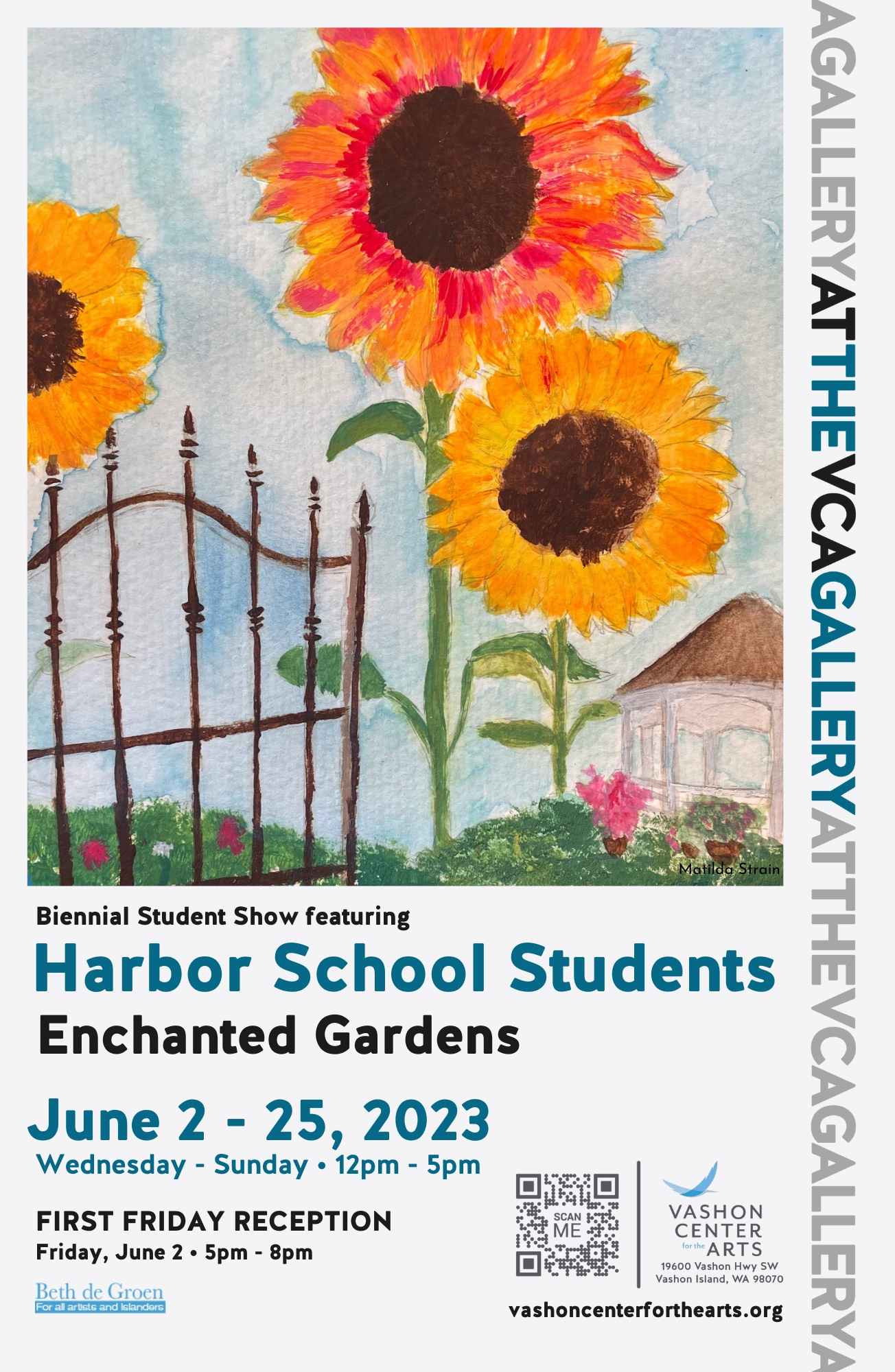This detailed advertisement for the Biennial Student Show at the Vashon Center for the Arts (VCA) features a student painting prominently on the top left third of the poster. The painting captures three large sunflowers beside a metal fence, with green grass and smaller flowers at the base. A distinctive pink house with a brown roof appears in the bottom right corner, along with the artist's name, Matilda Strain, in black lettering. The background includes lush green gardens, evoking the Channing Gardens where the event will be held from June 2nd to June 25th, 2023. The exhibition is accessible from Wednesday to Sunday, between 12 p.m. and 5 p.m., with a special First Friday Reception on June 2nd from 5 p.m. to 8 p.m. The right side of the poster repeatedly states "A Gallery at the VCA Gallery," emphasizing the hosting venue—the Vashon Center for the Arts, located at 19600 Vashon Highway Southwest, Vashon Island, Washington, 98070. A QR code marked "Scan Me," alongside the VCA's logo and URL (VashonCenterForTheArts.org), invites further exploration. The poster's color scheme primarily includes white, black, blue, yellow for the sunflowers, and green for the garden background.